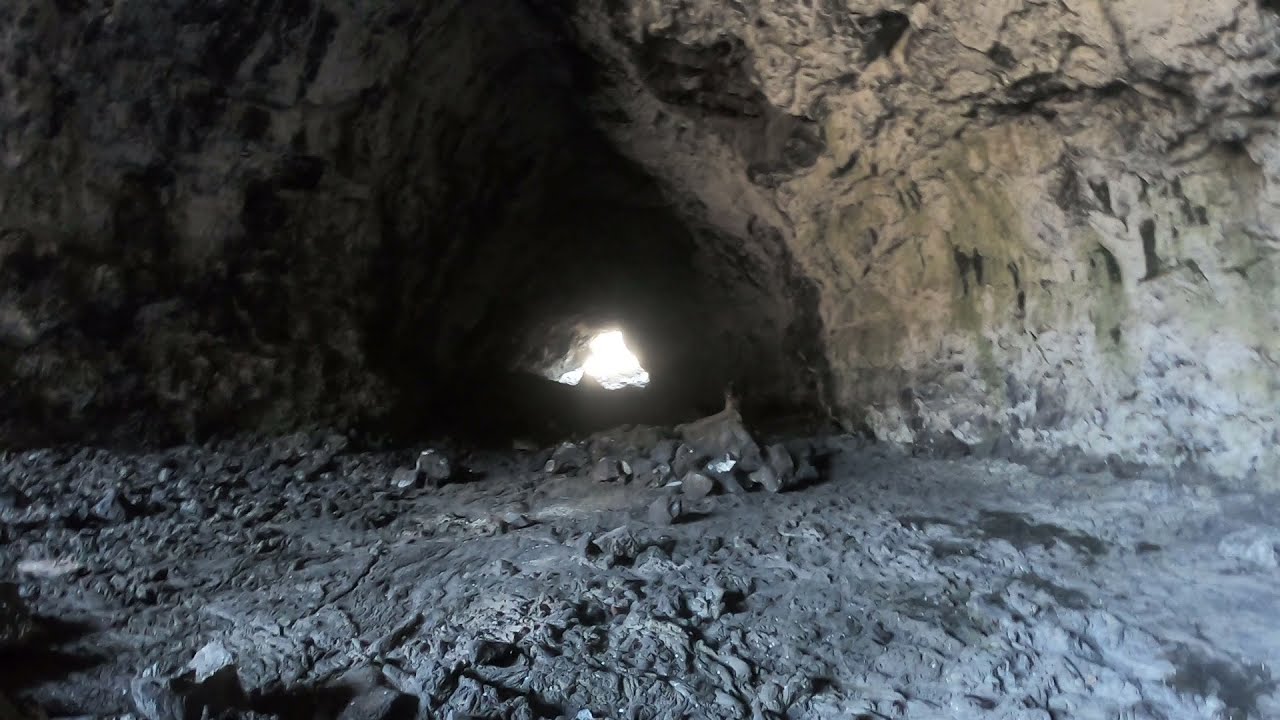The image captures the desolate interior of a cave, depicted in a horizontally aligned rectangular photo. The floor, covered with numerous small, gray, and dusty rocks, presents a rough, uneven terrain. The cave's walls, textured with hues of gray and white and marred by green splotches, rise from both the top left and top right corners, arching to create a dome-like structure. They converge towards the center to form a small, triangular tunnel. This tunnel leads to a bright, irregularly shaped hole that allows a flood of white light to pour in, creating an illuminated triangle that obscures any further view. Shadows cast by the rocks populate the bottom left of the image, further emphasizing the lonely and untouched nature of this cavernous space. No signs of life or movement are present, reinforcing the silent isolation within this rocky abode.